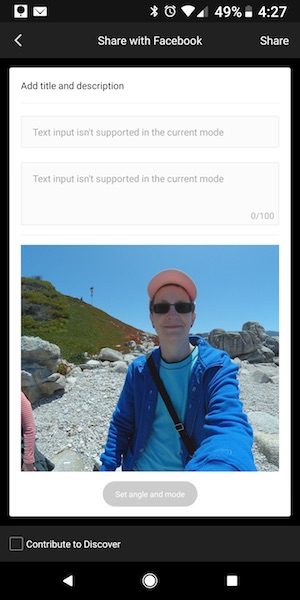This detailed caption represents a screenshot from a Facebook page:

"The image is a screenshot of a Facebook page interface encapsulated in a black border about an inch from the top and bottom edges and slightly smaller from the sides. The central part of the interface is white, providing a distinct contrast. 

In the top left corner, there is a series of icons: a square camera icon, followed by an email icon. To the right of these icons, the status bar displays various elements - the time '4:27', a battery icon at 49% charge, an Internet connectivity indicator, a full Wi-Fi signal, an alarm clock icon, and a Bluetooth icon.

Below the camera icon, a white greater-than sign points to the left. Centrally positioned on the screen is the text 'Share with Facebook', with 'Share' displayed on the right side. Directly beneath this text, the content divides into two sections. The upper half remains white, while the lower half features an image of a woman on a beach. The beach extends diagonally from the right side, with visible rocks and a small stretch of water. The background transitions from white to green about an inch from the top.

The woman is seen wearing a pink hat and sunglasses, looking straight ahead. She is dressed in a light blue shirt under a dark blue jacket, with a black strap of a pocketbook slung over her left shoulder and hanging down her right side.

In the white space above this image, there are editable fields labeled 'Add title and description'. Further down, still in the white area, there's a light gray tab reading 'Set angle and mode', followed by another section with a light gray square labeled 'Contribute to Discover'.

At the bottom center of the screen, three white icons are aligned: a circle in the middle, a square to the right, and a left-pointing triangle (formerly described as square) to the left, completing the interface depiction."

Feel free to adjust it to your preferred level of detail.